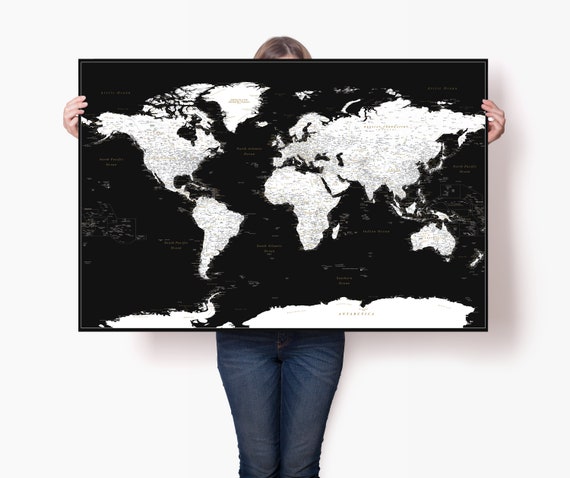The photograph features a woman standing against a solid white wall, partially obscured by a large rectangular map of the world which she is holding up with both hands. Her light-colored skin and medium brown to dark blonde hair are visible at the top of her head, while her torso is hidden behind the map. She is dressed in blue jeans, and her fingers, which are painted white, grasp the edges of the map. The map itself is black and white, with white continents labeled with gold or yellow text and black oceans. This setting gives the image a generic and adaptable appearance, hinting that it is likely used for displaying interchangeable visual products, such as custom artwork for online listings.